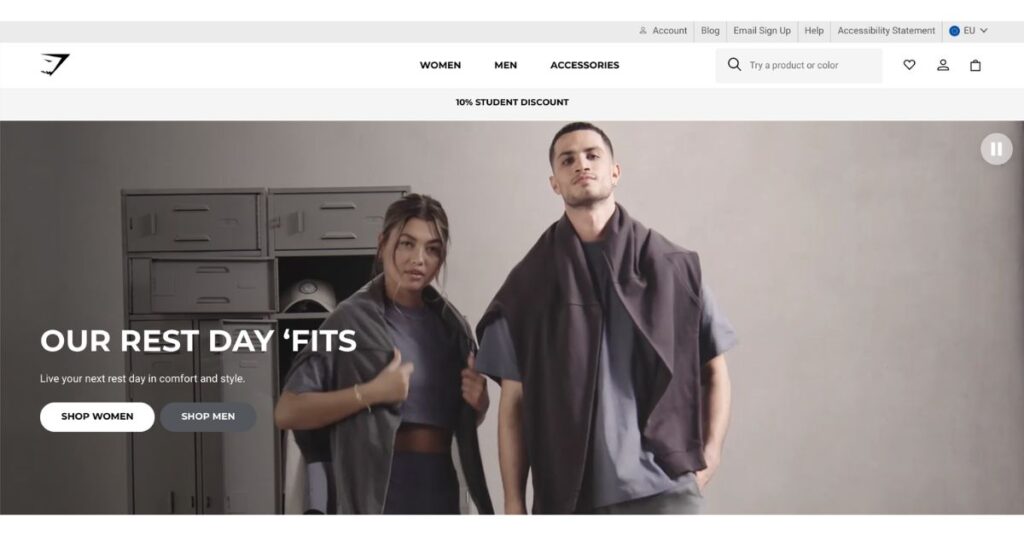**Descriptive Caption:**

The image displays a web page for a clothing brand emphasizing relaxed, comfortable outfits for rest days. The largest text on the page is in white and reads, "Our Rest Days Fits." Below this headline, a subheading states, "Live your next rest day in comfort and style." The background of the page is predominantly gray, featuring a gym-like locker. To the left, a woman is shown with a sweatshirt draped over her shoulders, revealing her midriff and dressed in a gray t-shirt and gray pants. To her right, a taller man stands with a similar sweatshirt over his shoulder, also wearing a gray t-shirt and gray pants. At the bottom of the page are two buttons: "Shop Women" in white and "Shop Men" in dark gray, directing users to browse the respective clothing collections.